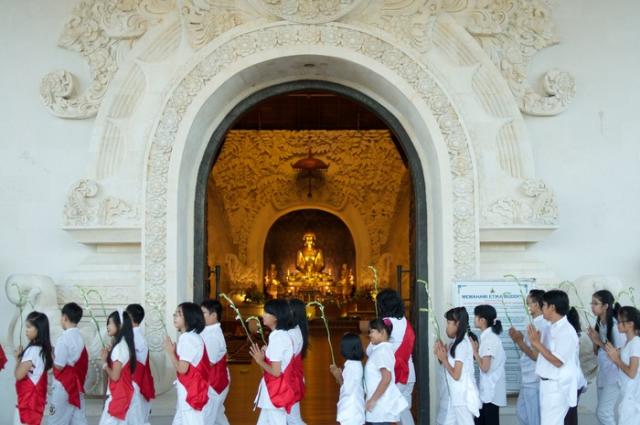This photograph captures a ceremonial procession outside a temple, likely situated in an Asian country, possibly Southeast Asia. The visual centerpiece is a magnificent white archway adorned with intricate carvings and Asian symbolism. Through this archway, there is a glimpse of a golden Buddha statue, placed amidst dim lighting and framed by more ornate decorations and smaller statues. The Buddha is under a bronze umbrella, contributing to the rich gold hues within the temple's interior.

In the foreground, the image features a group of children marching from right to left in two orderly lines. The children, who appear to be elementary-aged, possess uniform dark hair and are dressed in coordinated white attire. A notable distinction is observed in their attire: children on the left side wear red sashes, whereas those on the right side are in plain white clothing. The girls among them may be wearing white pants while boys have black pants. Each child holds a green stem or plant in a prayer-like position, suggesting a reverent, solemn atmosphere indicative of a structured religious procession. The children's expressions are serious, underscoring the significance of the occasion.